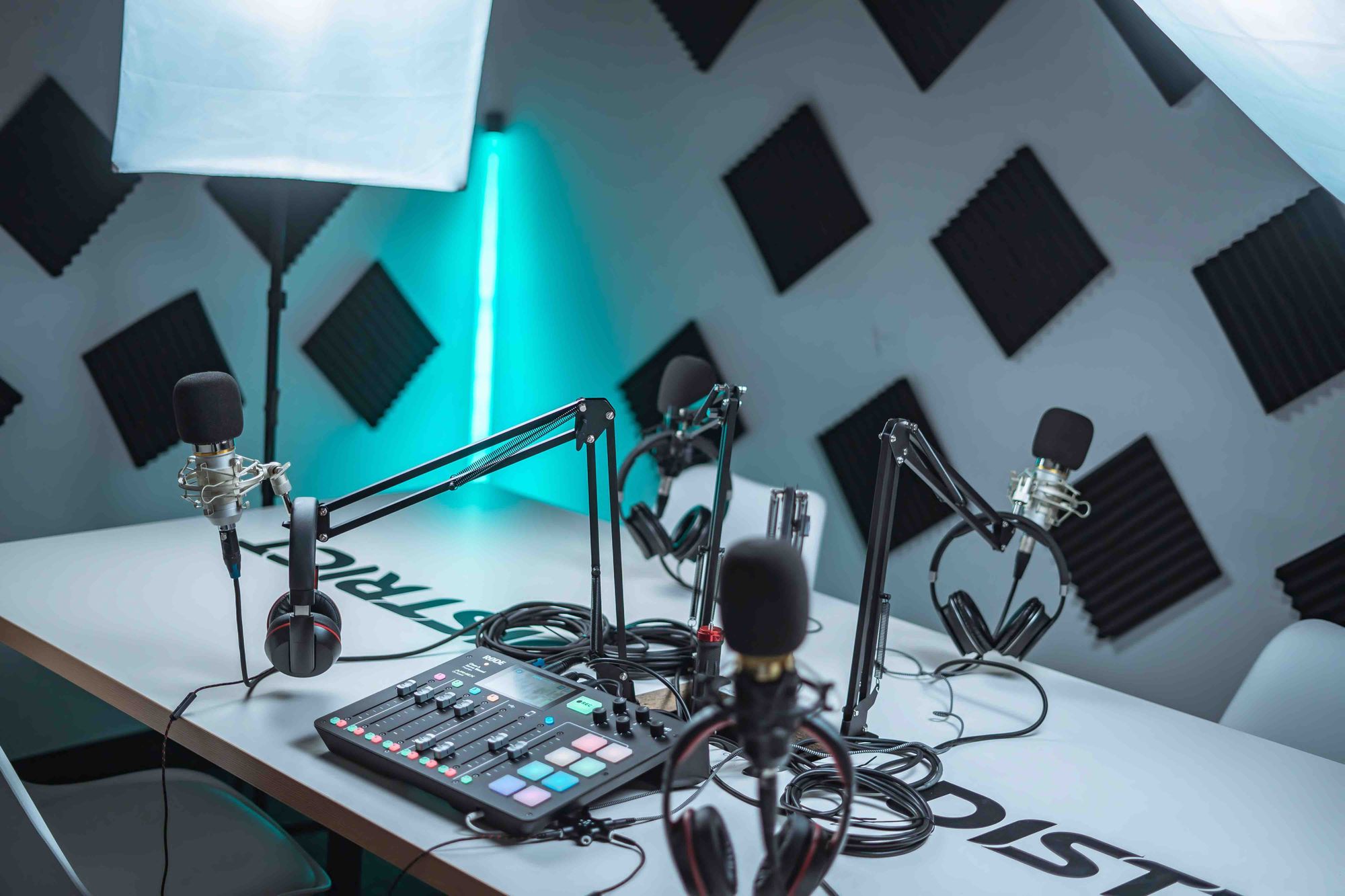The photograph depicts an elegantly constructed recording studio, characterized by its meticulous setup and modern equipment. The studio's white walls are adorned with black, corrugated foam squares strategically placed for soundproofing. Dominating the space is a large white table, equipped with a small sound mixing board and an array of four black microphones, each accompanied by over-the-ear headphones. The microphones are likely configured for podcasts or interviews, as suggested by the seating arrangement: two chairs situated on one side of the table and an additional chair visible on the opposite side, with room for a probable fourth. Illuminating the space are two large white lights, including a photography light with a square reflector, enhancing the room's visual clarity. In the background, a slender blue fluorescent light casts a soft glow, adding a modern aesthetic touch. The table itself bears a partial business name or logo that reads "district," with the text appearing to be oriented based on the viewer's position. The overall arrangement and equipment suggest a professional environment designed for high-quality audio recording and media production.